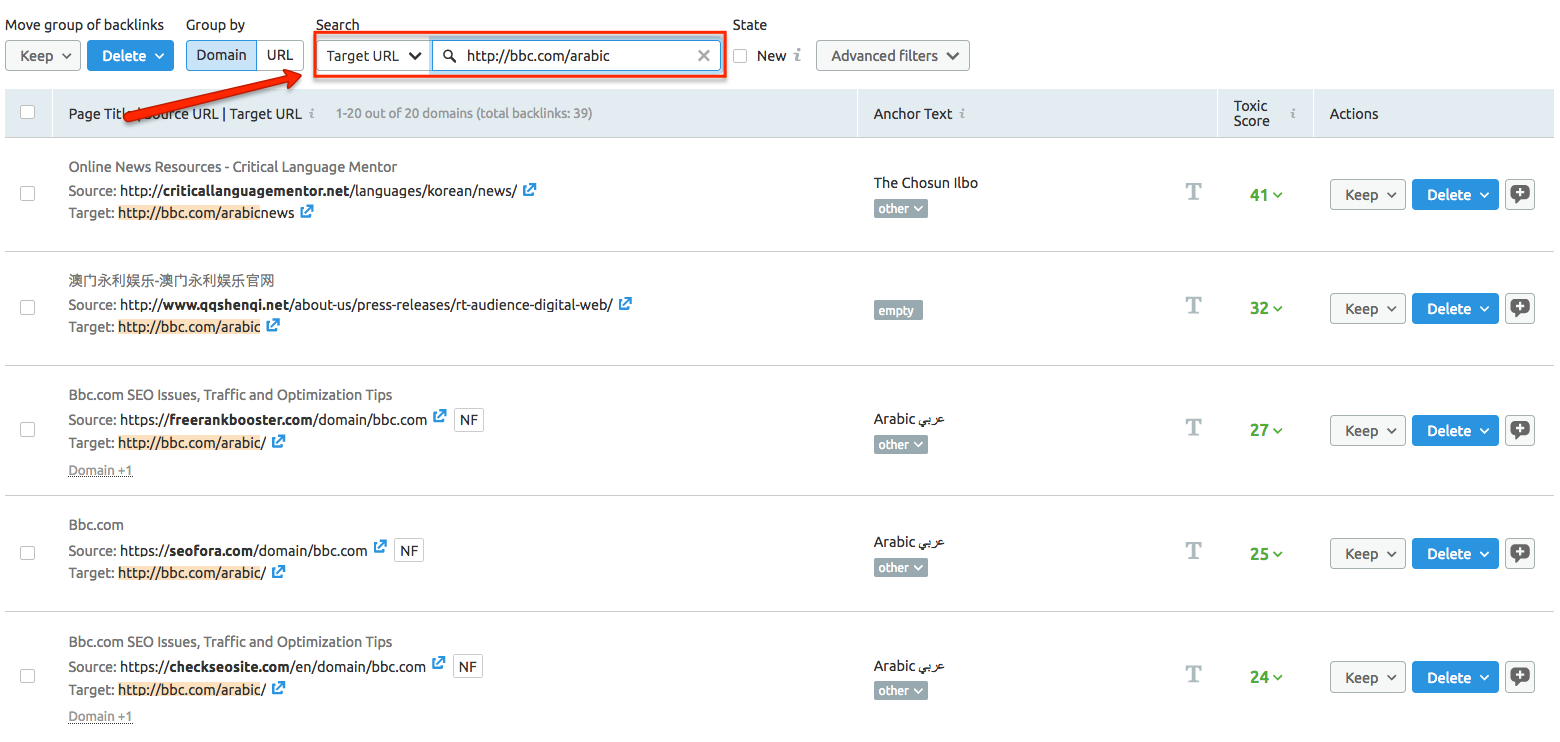This is a cropped screenshot of an admin panel specifically designed for managing backlinks to BBC articles. The image captures five entries listed on the page. At the top left corner of the panel, "Move group of backlinks" is displayed in very small black font. Directly below this text, there are two drop-down boxes; the left one reads "keep" and the right one reads "delete," with "delete" highlighted in blue. To the right of these drop-down boxes is a "Group by" section featuring two clickable options: "domain" and "URL." The "domain" option is currently selected. Further to the right, there is a search box flanked by another drop-down box on the left, which has "target URL" selected. Inside the search box, the text reads "BBC.com Arabic." Both the "target URL" drop-down and the adjacent search box are highlighted with a red box, and a red arrow has been edited into the screenshot pointing directly at "target URL." Below these elements is the list of articles, making this an instructional screenshot that demonstrates how to input a target URL in the search bar, select the corresponding option, and search for the specific website you wish to edit.